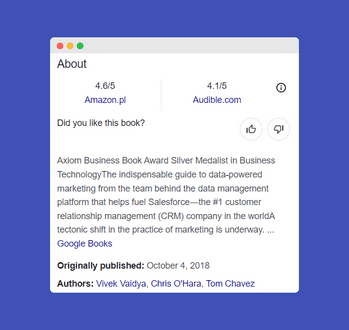This image is a screenshot taken from Amazon's website. The main focus of the screenshot is a promotional box with a distinct color theme. The outer layer of the box is primarily a shade that oscillates between purple and blue, creating a visually engaging border. Within this colored perimeter, there is a white square with a gray top edge. The gray section contains identifiable branding information, including 'amazon.pl' and 'audible.com', indicating its source.

Inside the white square, specific book details are provided, although the actual title of the book is not visible in this capture. Below the gray banner, there is information about the book's authors, listing three different writers. The original publication date is also noted, marked as October 4, 2018. Additionally, the book has received an accolade, specifically the Axiom Business Book Award Silver Medal in the Business Technology category, which is prominently mentioned within the box.

Towards the bottom of the box, there's a section prompting user interaction, asking if people liked the book with options to give it a thumbs up or thumbs down. Moreover, the book's rating is displayed, providing users with an overall assessment of its reception.